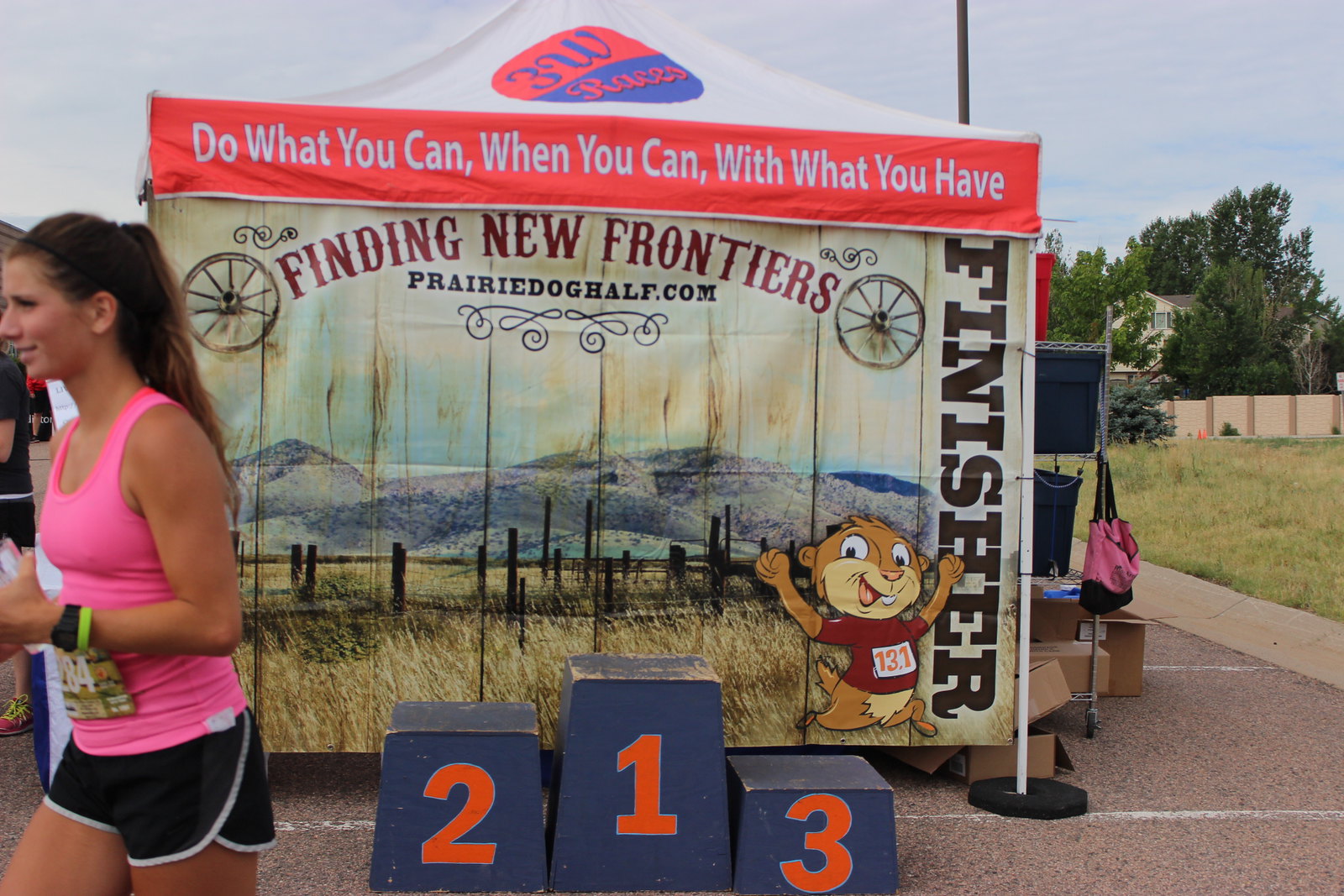The image captures what appears to be the end of a charity race set in an outdoor venue. Central to the scene is a first, second, and third place podium with large, dark gray blocks labeled 2, 1, and 3 in fluorescent orange. Prominently situated toward the left of the image is a brunette woman with brown skin, dressed in a fluorescent pink tank top and black dolphin running shorts. She is moving in a slow running or walking position, facing leftward. The woman also sports a wristband that's yellow and black. 

Behind the podium and the woman, there is a white canopy covered partially by a vibrant, fluorescent orange banner. The banner features a motivational quote in white text: "Do what you can, when you can, with what you have." Below this, a prairie-themed visual includes two brown wagon wheels flanking the phrase "Finding New Frontiers" written in old-timey red letters, followed by the website PrairieDogHalf.com in black lettering. On the bottom right of the banner, a cartoon prairie dog raises its arms triumphantly, wearing a shirt emblazoned with the number 131. This section of the banner is accompanied by the word "Finisher" running vertically along the right side.

The background behind the canopy showcases a scenic mountain range with a brown field and fence in the foreground, completing the prairie theme. To the right of the banner is a grassy area surrounded by trees, indicating the outdoor, natural setting of the event. Additionally, there's a piece of luggage hanging off the right edge of the canopy, resting on what appears to be concrete pavement.